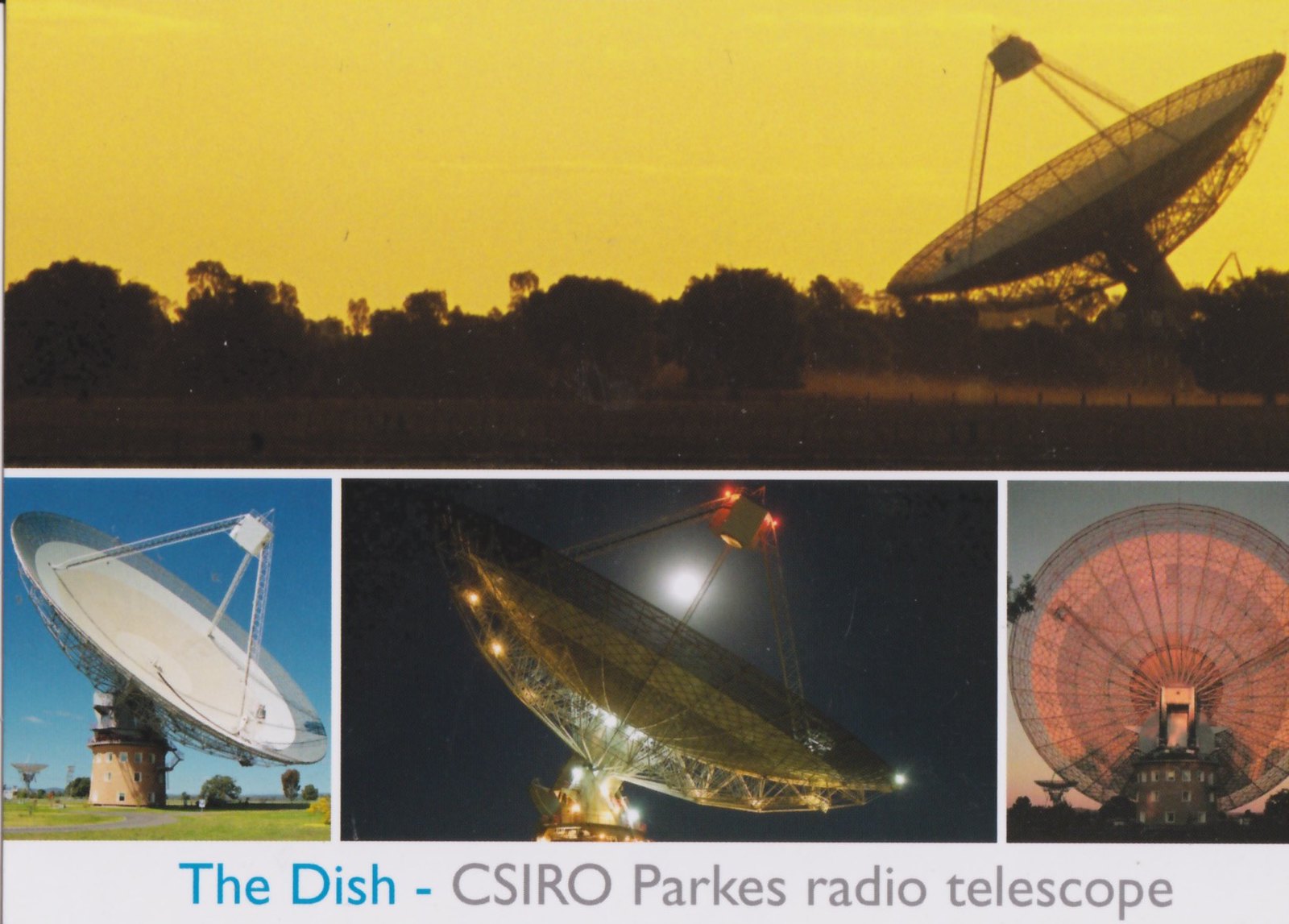This image is a collage titled "The Dish CSIRO Parkes Radio Telescope," with four photographs showcasing the large satellite dish in various settings and times of day. The primary top image spans the width of the collage and captures the telescope in silhouette against a striking yellowish sky during sunset, with tree outlines in the background. Below, on the left, a daytime shot displays the dish in a green grass field against a clear blue sky, pointing to the right. The center bottom photograph highlights the dish at night, illuminated with its lights on, with the moon visible in the distance. The bottom right image, taken from behind the dish at either dawn or twilight, features a soft, pinkish-orange sky, reminiscent of a Ferris wheel from this angle. The repeated text at the bottom confirms the subject as "The Dish CSIRO Parkes Radio Telescope," emphasizing the iconic structure's various atmospheric and temporal contexts.